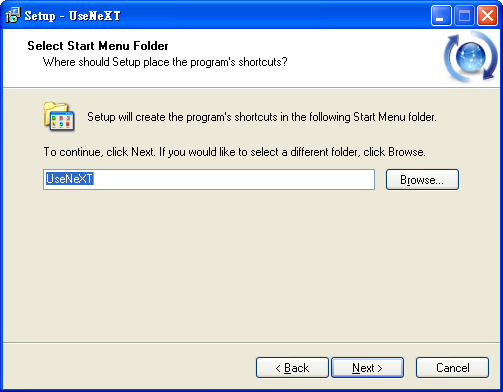This image depicts a screenshot taken on a Windows XP computer, featuring a setup dialog box for the installation of a program called UseNext. The entire background is a solid white, and the pop-up window dominates the center of the image. The dialog box is headed with "Setup - UseNext" and prompts the user to "Select Start Menu Folder," asking where the program shortcuts should be placed. The instruction text below reads, "Setup will create the program shortcuts in the following Start Menu Folder. To continue, click Next. If you would like to select a different folder, click Browse."

In the screenshot, the program name, "UseNext," is pre-filled in a text field which is highlighted in blue. Adjacent to this field is a "Browse" button, allowing the user to select a different folder if desired. The bottom section of the dialog box includes three interactive buttons: "Back," "Next," and "Cancel," each set against a typical grayish-brown background. The screenshot features a combination of colors including blue, white, red, yellow, orange, gray, and tan, which contribute to the traditional Windows XP style and functionality.